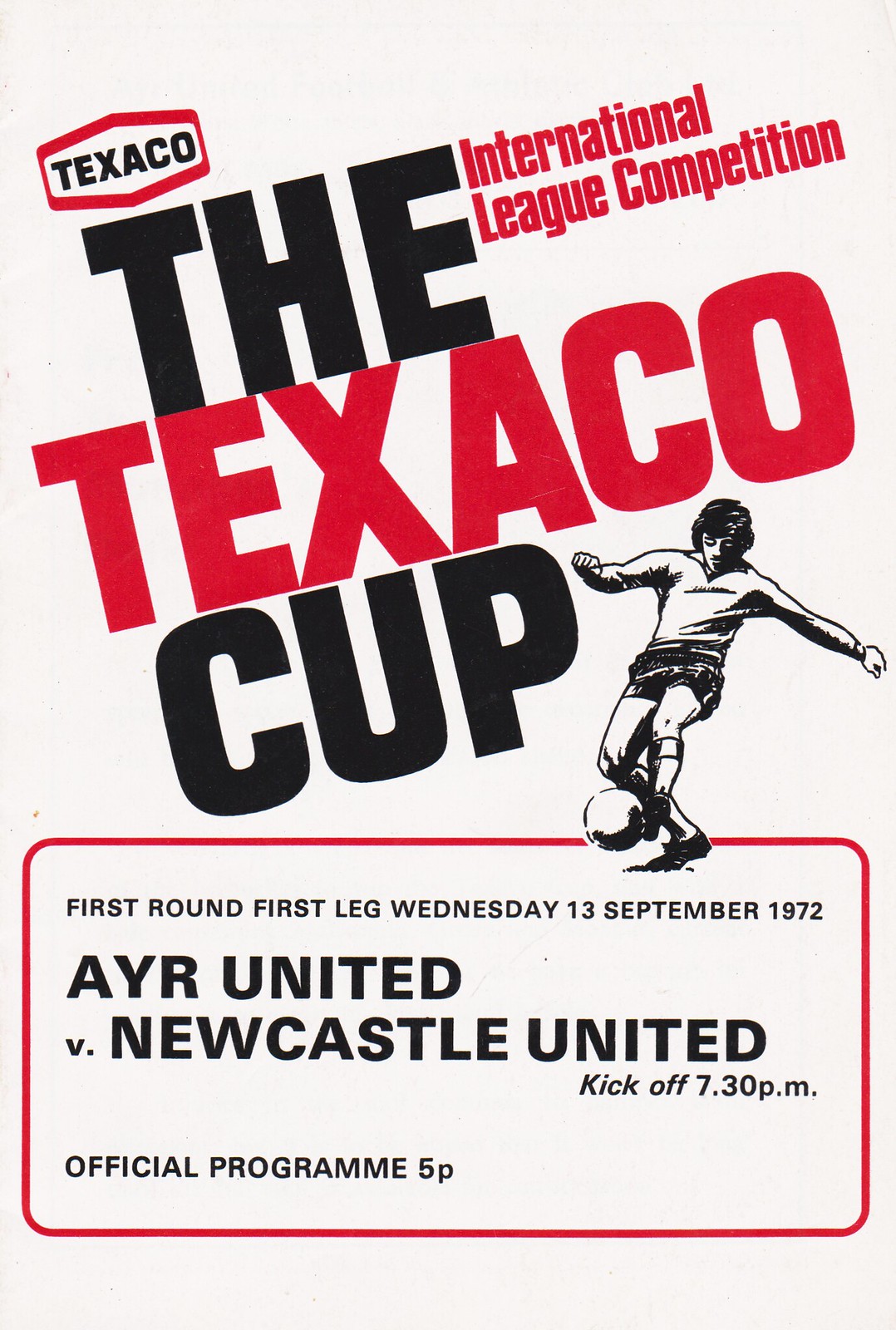This is the front cover of a football program for the International League Competition Texaco Cup. The background is white, with large, bold, uppercase text in black and red. In the upper left corner, there is a Texaco logo. Centered at the top, in alternating black and red text, it reads "International League Competition Texaco Cup." To the right, there is a black-and-white drawing of a man kicking a soccer ball. Below this, a red rectangle with rounded corners frames additional details: "First Round, First Leg, Wednesday, 13 September 1972." Below this, in more prominent text, it announces "AYR United vs. Newcastle United," with the kickoff time at 7:30 PM. The bottom of the rectangle notes "Official Program 5p".